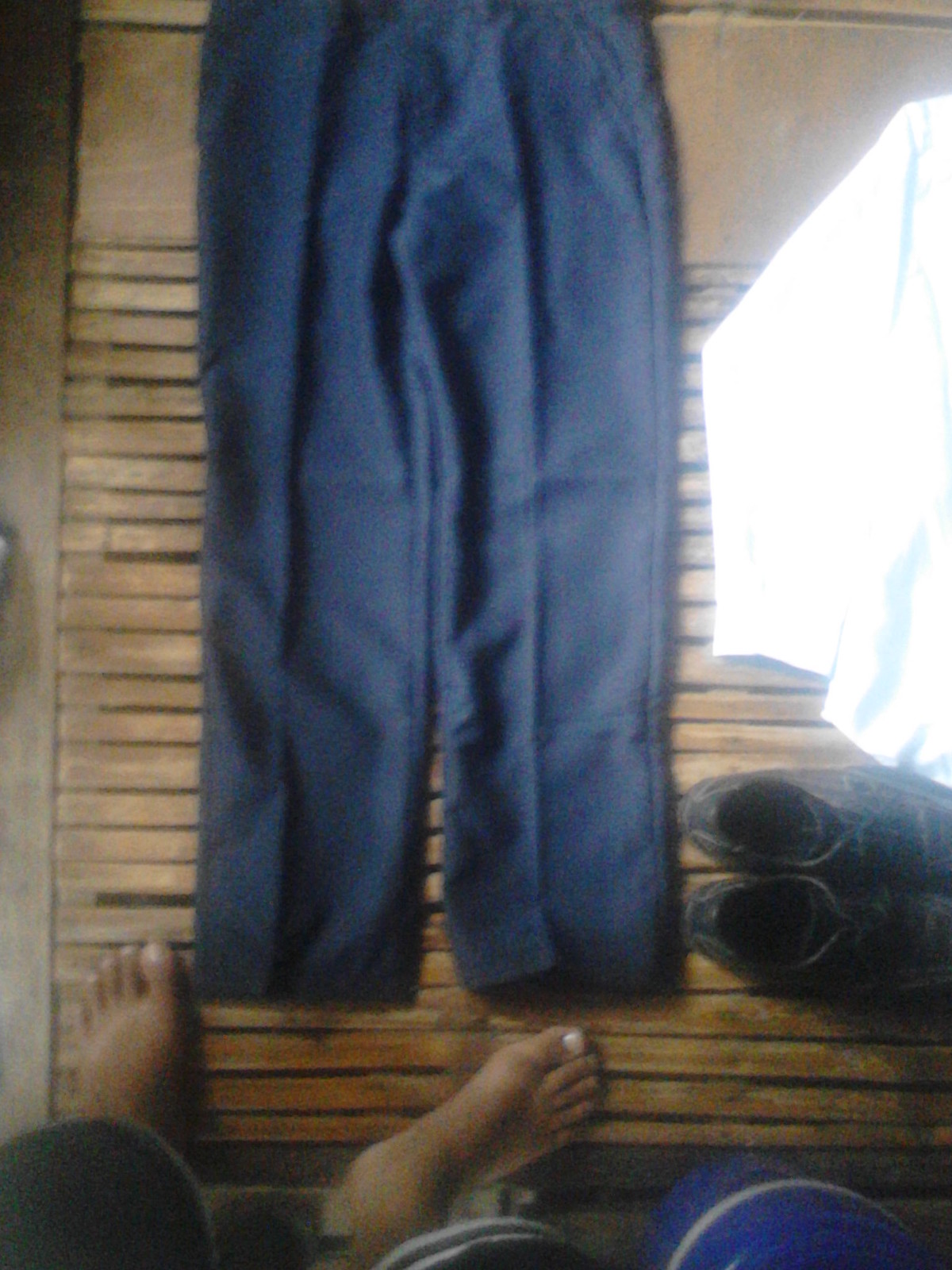A blurry photograph appears to be taken from a cellular device, capturing a scene from above. In the center of the image lie a pair of blue-black slacks, positioned vertically on wooden flooring with horizontal slats running left to right. The pants seem slightly wrinkled, suggesting a casual placement. In the bottom left corner of the image, the photographer's feet are visible, standing on the wooden surface. To the right of the feet, there's a pair of brown or perhaps black men’s shoes, and partially captured on the right side of the image is the left half of a white-collared button-up shirt. A blue bucket is also visible near the top of the photograph. The entire scene is illuminated brightly, contributing to the overall blurriness and making detailed observation slightly challenging.